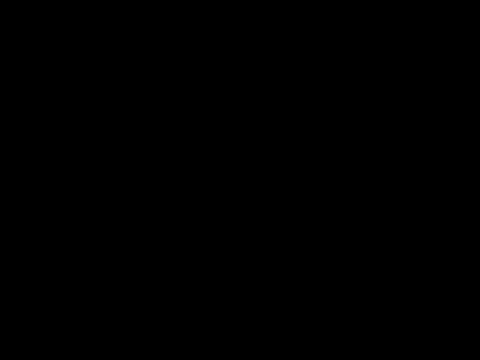The image is a plain black rectangle, slightly wider than it is tall. There are no visible colors, shapes, text, or hidden images—just a solid black surface with no variation or detail. The entire image is composed of uninterrupted blackness, making it appear as though it is a simple void.